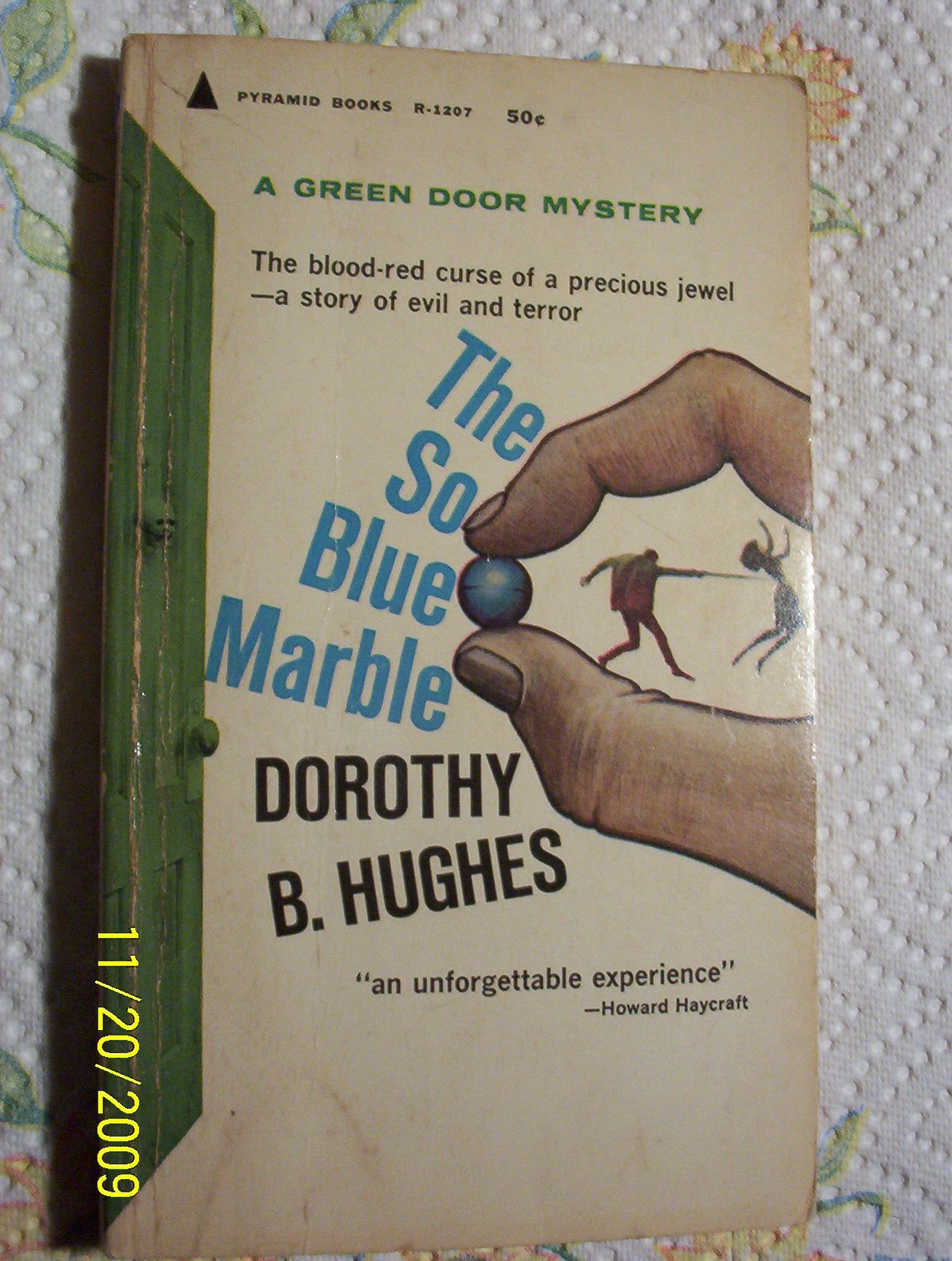This detailed portrait-mode photograph, timestamped 11-20-2009, features the cover of an old, off-white hardback book with a green binding. The book, titled "The So Blue Marble" by Dorothy B. Hughes, is situated on a quilted paper towel adorned with green leaves and yellow flowers. Prominently at the top of the cover, a black triangle contains the text "Pyramid Books R1207" and indicates a price of 50 cents. Adjacent to it is the phrase "A Green Door Mystery," which is inscribed in green lettering. Below that in black text, it reads "The Blood Red Curse of a Precious Jewel - A Story of Evil and Terror".

The upper right of the book cover features an illustration of a hand where an index finger and thumb pinch a blue marble. Within the circular space created by the fingers, a vivid image depicts a man in brown holding a sword aimed at a woman in a blue dress. To the left of the hand, the title "The So Blue Marble" is written in blue text, and below it, the author's name, Dorothy B. Hughes, appears in black print, alongside the endorsement "An Unforgettable Experience" by Howard Haycraft.